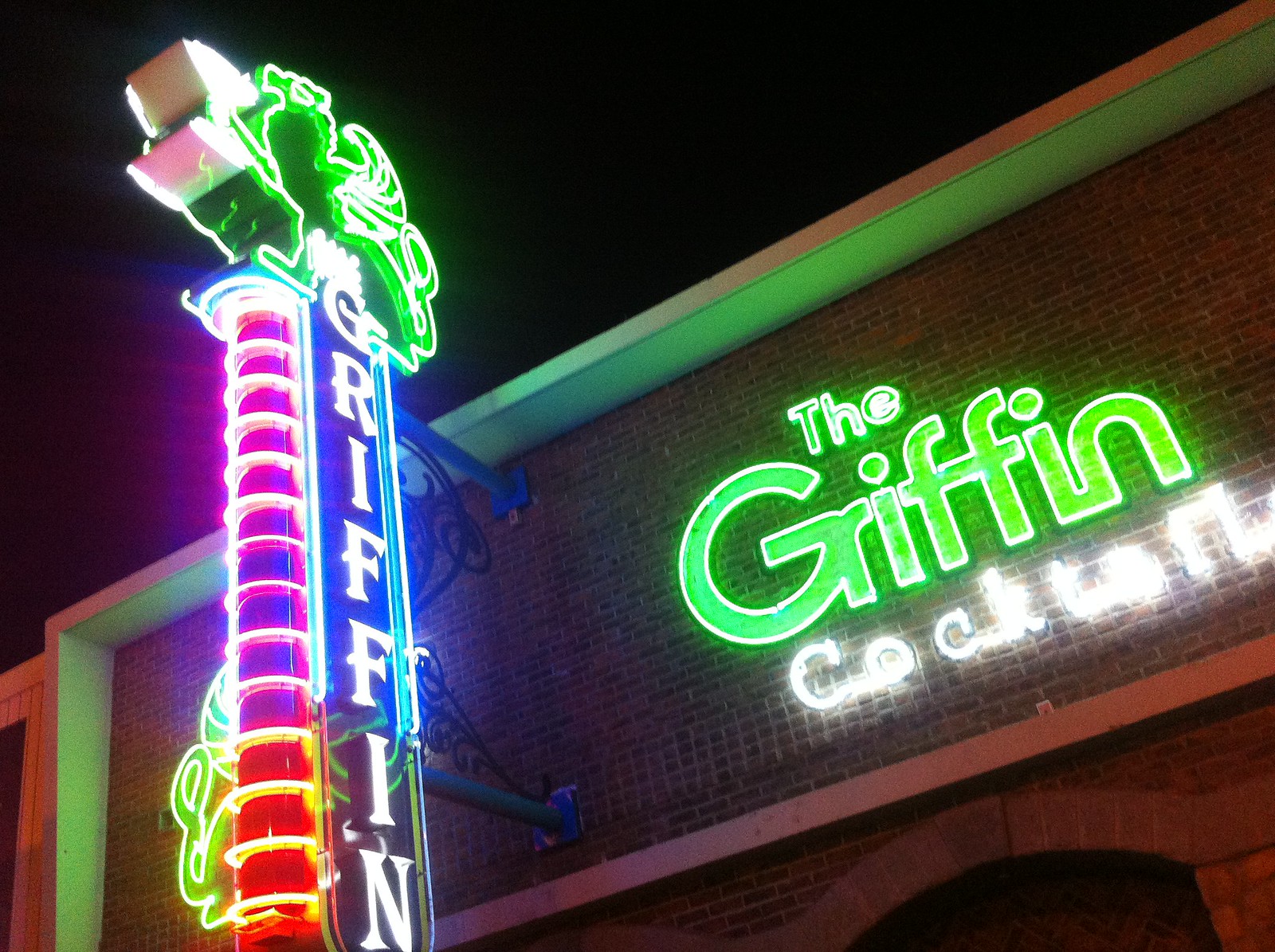The image captures an almost perfectly square photograph taken at night outside a bar or club, featuring a prominent brick wall with a white border at the top. Centered on the wall, there is a green neon sign displaying the words "the Griffin," with "the" in smaller letters and "Griffin" in larger letters. Below this, another neon sign in white letters reads "cocktails." To the left, hanging perpendicularly off the building, is a vertical neon sign with a green image at the top and the word "Griffin" vertically written in white. Surrounding the vertical sign are reddish-orange neon lines. The green image at the top of this sign, possibly a lion or an angel, extends slightly from the left side. The background behind the building reveals a stark, black night sky.